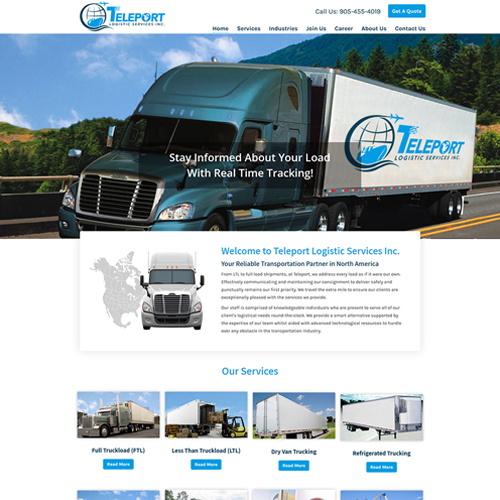This image is a detailed screenshot of the Teleport Logistics Services, Inc. website homepage. At the very top of the page, there's a header with a white background. Positioned towards the left side, the company name "Teleport" is prominently displayed in a light sky blue font, using capital letters with a significantly larger "T." Adjacent to the name is a simplistic drawing of a globe encircled, forming the company logo.

The header also includes a horizontal navigation menu listing the following items: "Home," "Services," "Industries," "Join Us," "Career," "About Us," and "Contact Us." On the right side of the header, there is a prompt to "Call us" followed by a phone number, along with a blue rectangle button that says "Get a Quote" in white text.

Beneath the header, a large photo showcases a truck on the road, with the company logo "Teleport" visible on the side of its white trailer. The truck's cab is painted in a striking aquamarine green color. The backdrop features a picturesque scene of blue skies and mountains, enhancing the visual appeal.

Below the main image, there is a rectangular section with a white background and a light gray outline. Inside this rectangle, the text "Welcome to Teleport Logistics Services, Inc." is written in blue. Directly underneath, a smaller gray text reads "Your reliable transportation partner in North America." Below this slogan, there is an unreadable gray text due to its small size. This section also includes an image of a truck viewed from the front, with a white cab, alongside a light gray map of North America.

Following this introductory section, there's a headline titled "Our Services," under which four photos of trucks are displayed. Each photo has a description underneath. However, only some descriptions are legible: the one on the far right reads "Refrigerated Trucking," and the one on the far left reads "Full Truck Load." The details under the remaining two photos are too small to decipher.